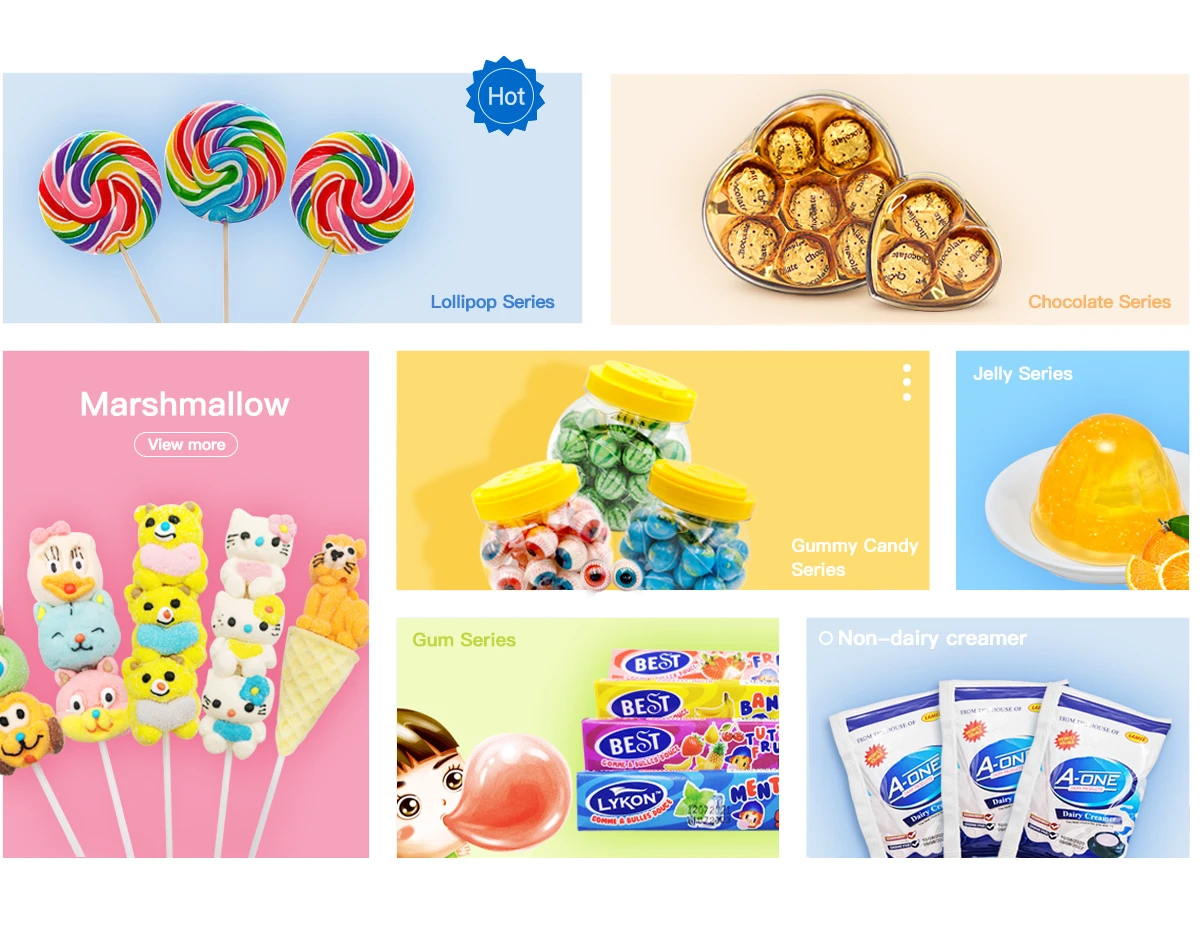The website displayed in the image features a vibrant and engaging mosaic layout consisting of seven distinct product categories. Each category is showcased within its own box, highlighting a different item for sale.

- **Upper Left Corner**: This box is dedicated to the "Lollipop Series," featuring an enticing trio of lollipops. The box is accentuated by a "HOT" label in the corner, indicating its popularity.
- **Upper Middle Right**: The "Chocolate Series" is displayed next, depicting two different boxes of delectable chocolates. 
- **Lower Left Corner**: Here we find the "Marshmallow" section. The image shows five marshmallow characters on sticks, accompanied by a "View More" option to explore additional varieties.
- **Middle Center**: Positioned in the middle is the "Gummy Candy Series," featuring three tubs topped with bright yellow lids.
- **Lower Middle**: Below the gummy candies is the "Gum Series." A playful cartoon kid is seen blowing a bubble, surrounded by four different bubblegum packages.
- **Lower Right Corner**: The "Non-Dairy Creamer" category is displayed with three packages of the product.
- **Middle Right**: Above the non-dairy creamers, we have the "Jelly Series," showcasing a selection of jello-like treats.

This carefully arranged mosaic provides a comprehensive and visually appealing overview of the assorted confectionery and related items available on the website.